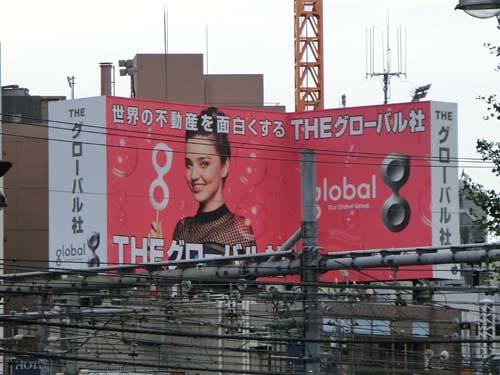In the image, there is a prominent red banner featuring the number 8, which appears to be part of a logo, along with Chinese characters. The banner also includes the word "Global" and another instance of the number 8. Positioned against a backdrop of numerous telephone lines, a red tower is visible, enhancing the busy, urban setting. Adjacent to the tower, there is a white section of the banner that also bears Chinese characters and the word "Global." The scene is set against a stark, plain white sky, which contrasts with the vibrant red of the banner and tower. In the background, several buildings contribute to the bustling cityscape.